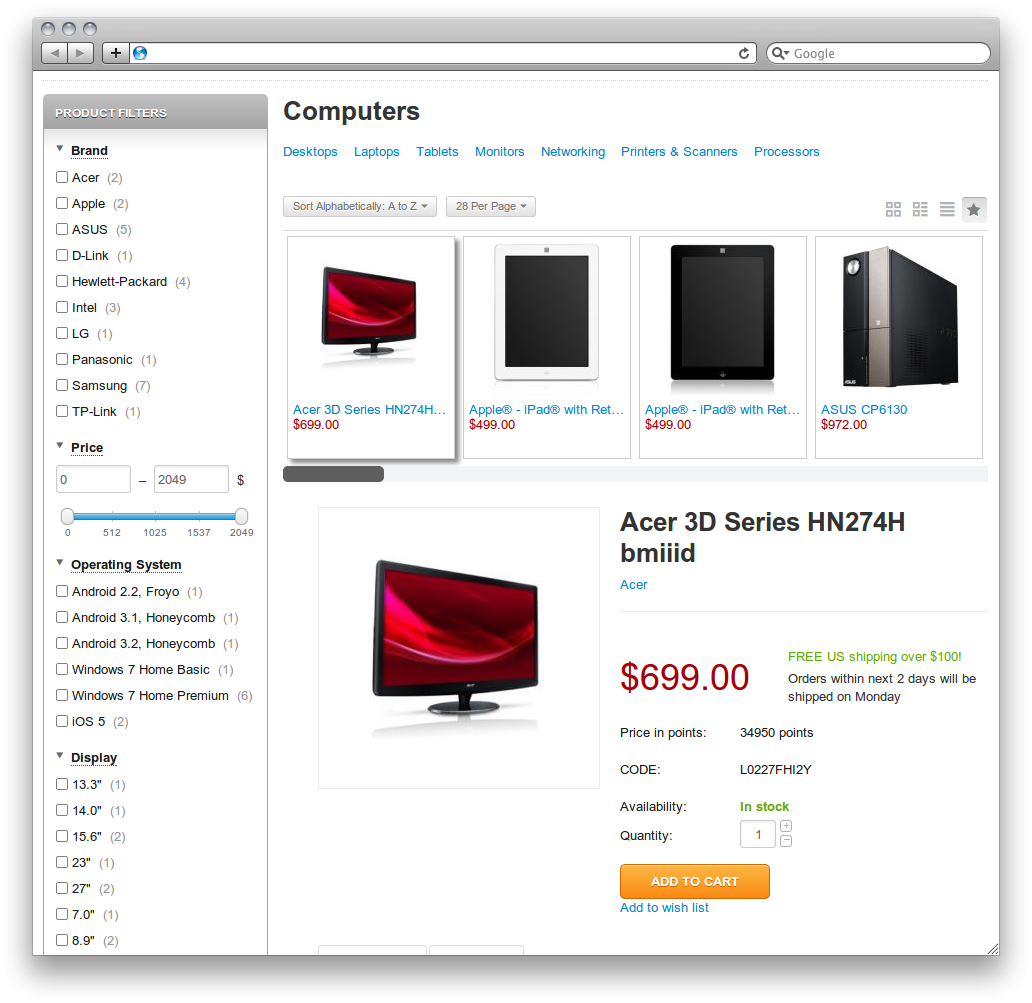**Detailed Caption:**

This vertical image captures a screenshot of a webpage displayed on a computer monitor. At the very top of the screen, there's a thin gray bar stretching horizontally across, featuring three gray circles on the upper left. Adjacent to this, there are back and forward arrows that are currently inactive, followed by a plus sign, a search bar with a refresh arrow beside it, and another Google search bar.

Below this toolbar, the webpage is divided into two main sections. On the left-hand side, there's a white background featuring a gray box labeled "Product Filters." This section allows users to filter products by various categories including brand, price, operating system, and display size. The filters for these categories have not been selected.

On the right-hand side, at the top of this section, "Computers" is prominently displayed in bold black text. Underneath, there are category options listed in blue: Desktops, Laptops, Tablets, Monitors, Networking, Printers & Scanners, and Processors.

Beneath these categories, two gray bars offer sorting options. One allows sorting items alphabetically, and the other provides the option to display 28 items per page.

The main content area showcases images of different types of computers. The highlighted product is the "Acer 3D Series HN274H BMI IID Acer," priced at $699. Below the product image, there is detailed information about the price, product code, availability, and quantity. Additionally, it offers free shipping. An orange "Add to Cart" button is prominently displayed, accompanied by a blue "Add to Wish List" option below it.